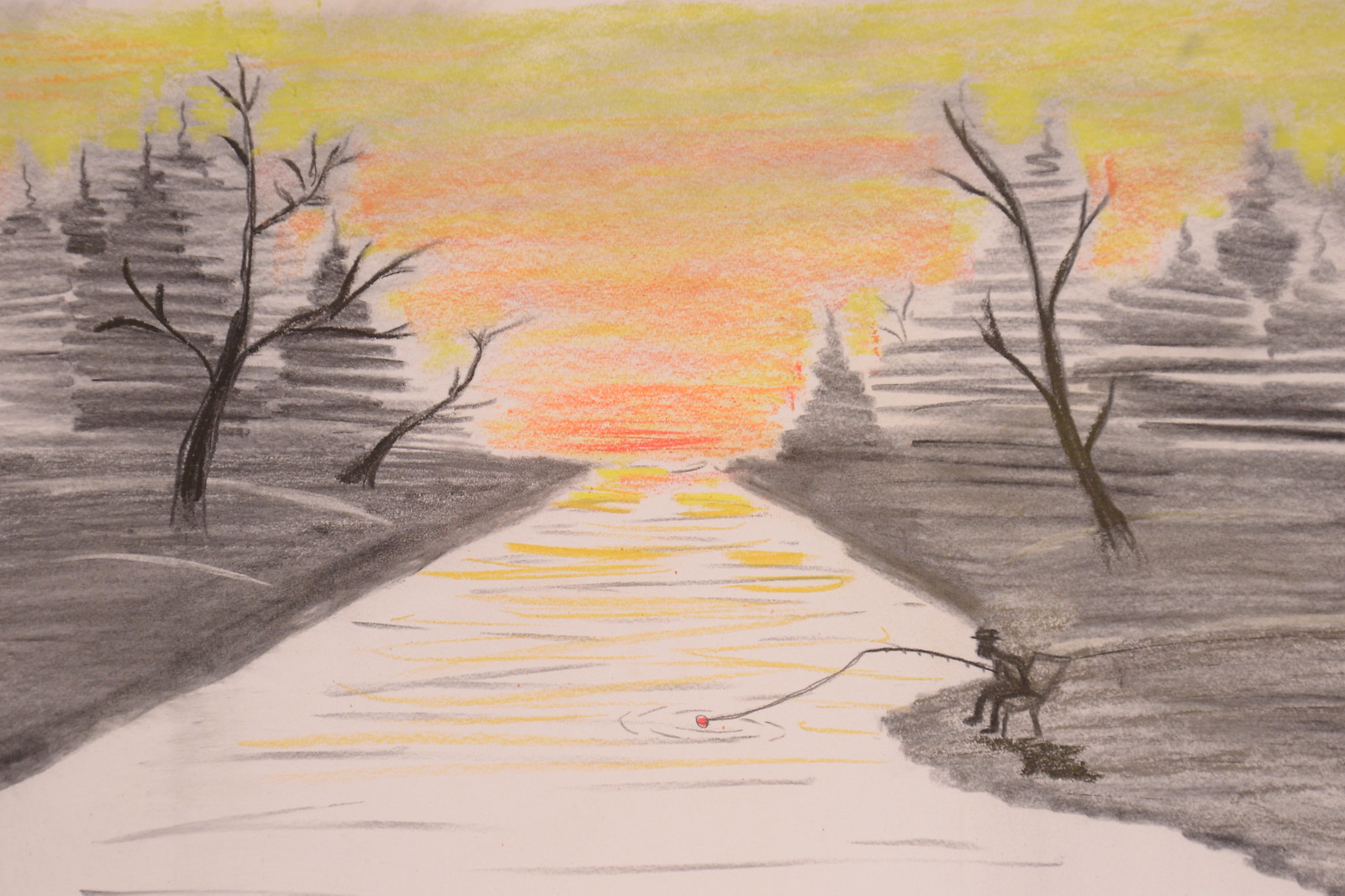This art piece is a sketch, likely created using chalks on paper. The composition features a serene river scene at sunset. The river originates from both bottom corners of the image and converges at the horizon line in the center, where it meets a vibrant sunset. The river itself is depicted in white, with dynamic grey and black lines illustrating the movement of the water. The backdrop of the setting sun utilizes a gradient of deep orange transitioning to pure yellow, enhancing the evening ambiance.

The riverbanks are rendered in dark grey, almost black, providing a bold contrast. The left bank is straight, while the right bank is curved. Nestled in the curved riverbank is the silhouette of a man seated on a chair, holding a fishing pole with its line cast into the water, surrounded by ripples near a float. At his feet lies an undefined object, adding an element of intrigue.

On the left riverbank stand two bare trees, with an indication of pine trees drawn behind them using simple horizontal lines forming pyramid shapes. The right riverbank mirrors this with a single leafless tree and additional pine tree silhouettes. This detailed depiction not only captures the natural beauty of the scene but also evokes a sense of calm and solitude as day turns to night.